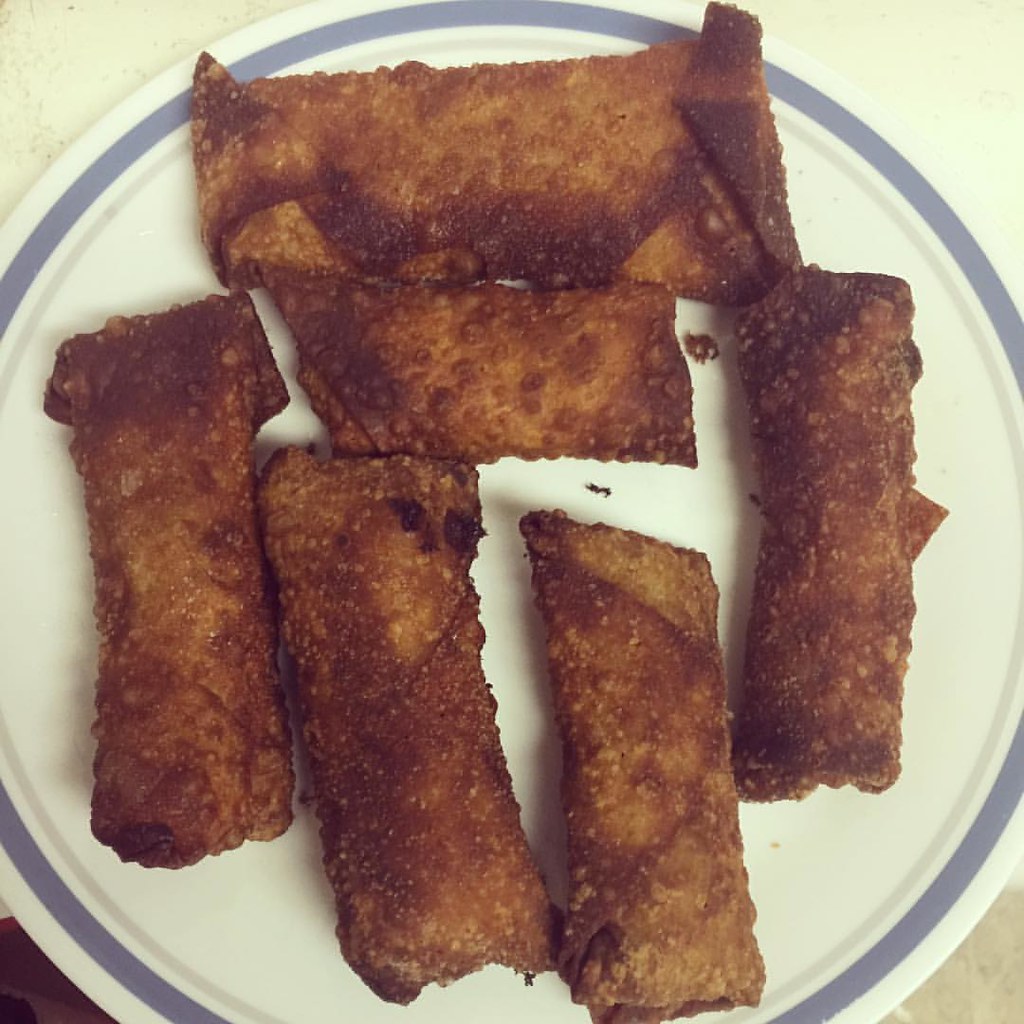This is an overhead view of a plate of homemade egg rolls, unmistakable due to their irregular folding and varied sizes. The egg rolls are deep-fried to an extra brown finish, with some crispy areas and flaking crumbs scattered on the plate. The plate itself is white with a blue border, possibly light purple, and it rests on a yellowish-white table or tablecloth. There are six egg rolls in total, four aligned vertically and two horizontally. The egg roll at the top, which is horizontal, looks the worst, resembling an envelope more than a conventional roll. The one on the far left is also poorly folded, with the top part looking haphazardly done. Despite their appearance, they appear to be freshly made, evidenced by the bubbling texture from the frying oil.